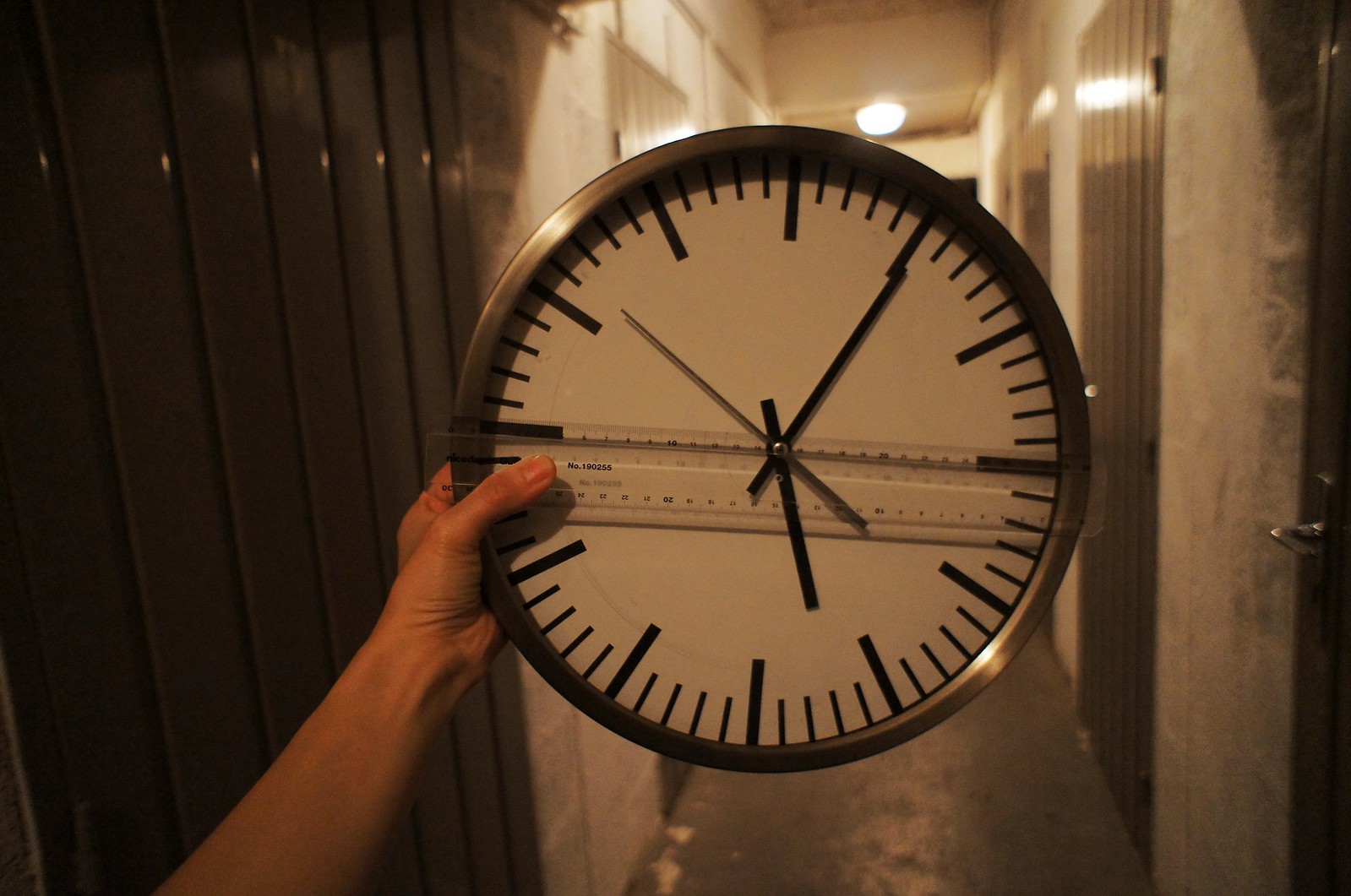In the photograph, a woman with fair skin is holding a large, circular analog wall clock up to the camera with her left hand. The clock features a coppery or metallic silver frame, and the face is white with black lines instead of numbers marking the hours, exemplifying a minimalist design. Positioned at 5:05, the black hour, minute, and second hands provide the current time. The woman's other hand holds a clear ruler across the clock for size reference, suggesting the clock's diameter is approximately one foot. The setting appears to be a conservative room, potentially an office or an apartment, with a plain decor and a hallway in the background.